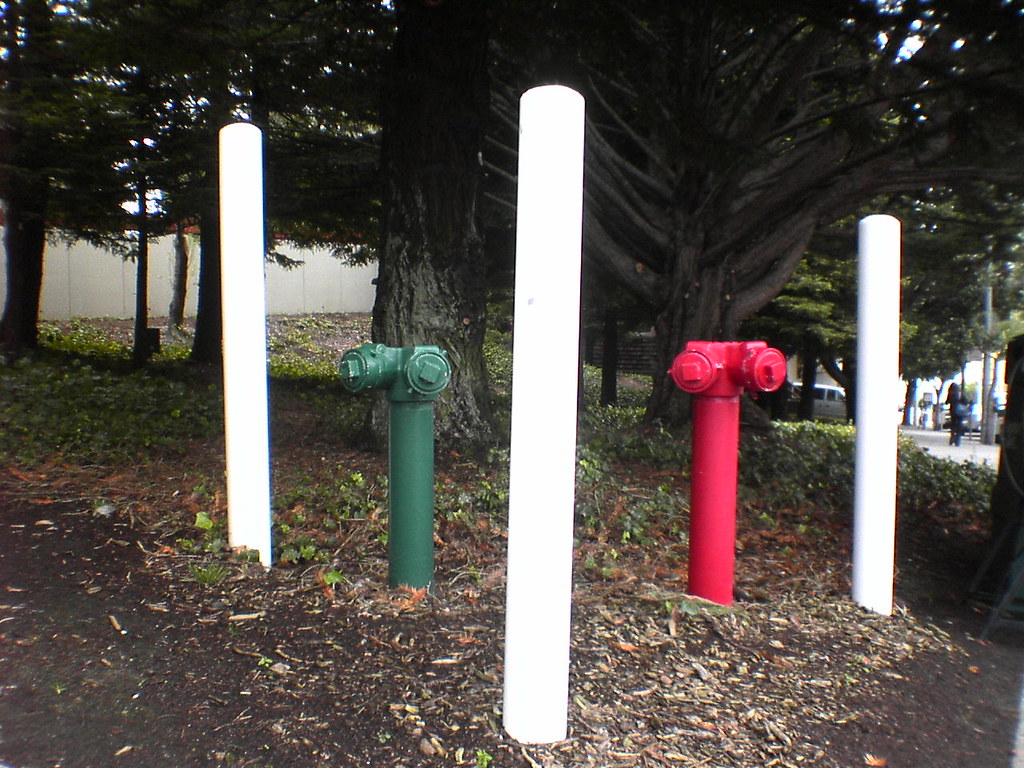The image captures a park-like area taken from the top of a hill, with a visible parking lot on the right and an SUV. A building can be observed on the left side. The foreground features a mix of dirt, leaves, pine straw, and debris covering the ground. Prominently, there are three white poles protruding from the ground, possibly made of metal or cement. In the middle, two vertical pipes, one green and one red, resembling fire hydrants or water pipe connections, stand at about half the height of the white poles. These colored pipes have bolts to open valves likely used for utility purposes. Trees across the background provide ample shade with scattered green grass around. A sidewalk, seen to the far right through an opening in the trees, hints at a person standing nearby, further emphasizing the park setting.